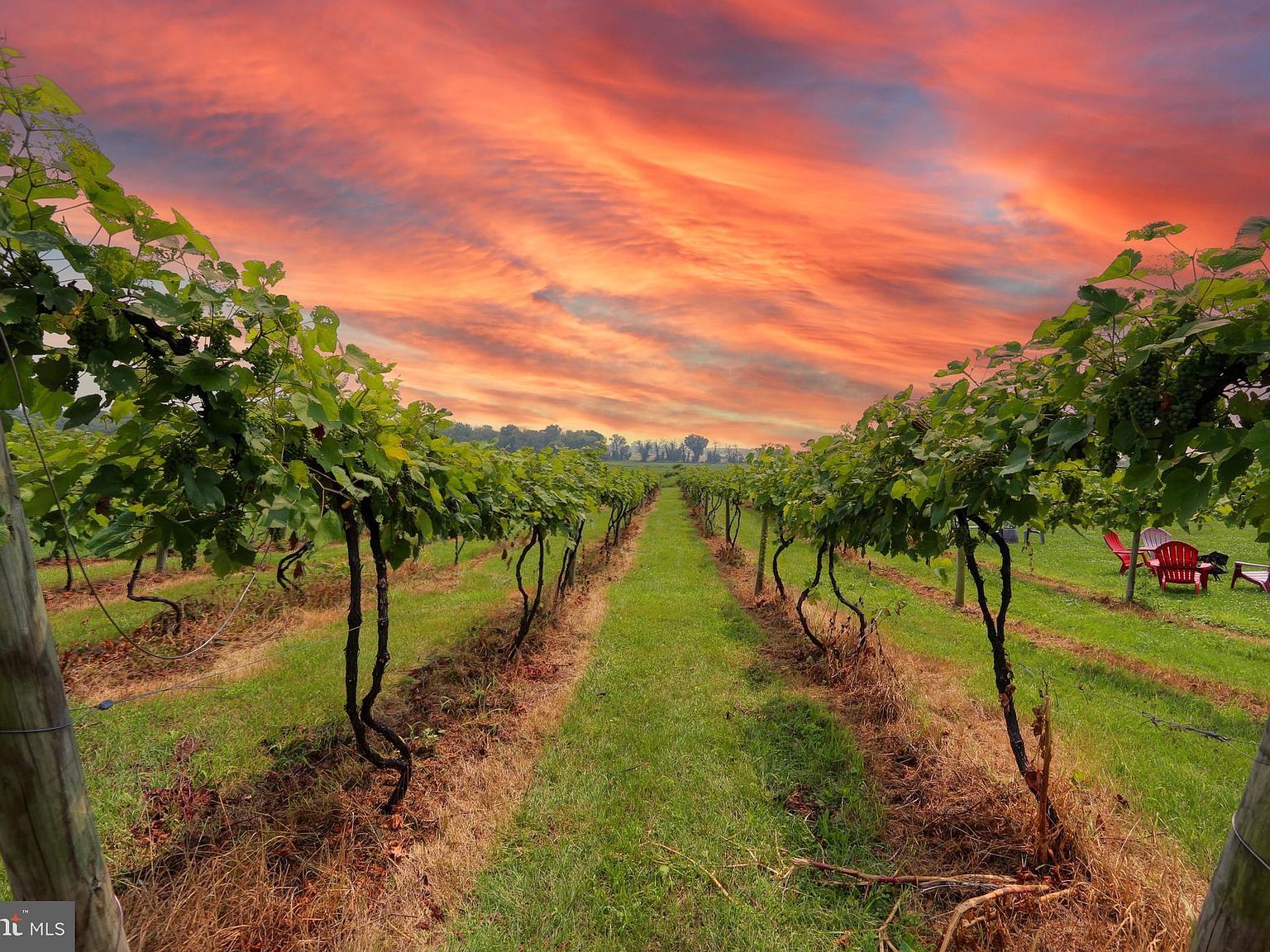This captivating outdoor scene captures a serene vineyard at either sunrise or sunset, casting a warm, inviting glow across the landscape. The sky is a stunning blend of pink, orange, and blue hues, creating a breathtaking backdrop. Stretching into the distance are meticulously arranged rows of grapevines, with slender, dark trunks and lush green leaves. The vineyard rows are separated by grassy trails, giving a sense of structured symmetry. On the far right, red Adirondack chairs are nestled in the grass, adding a charming touch to the peaceful setting. In the distance, the horizon is lined with trees, enhancing the picturesque quality of this tranquil vineyard scene.